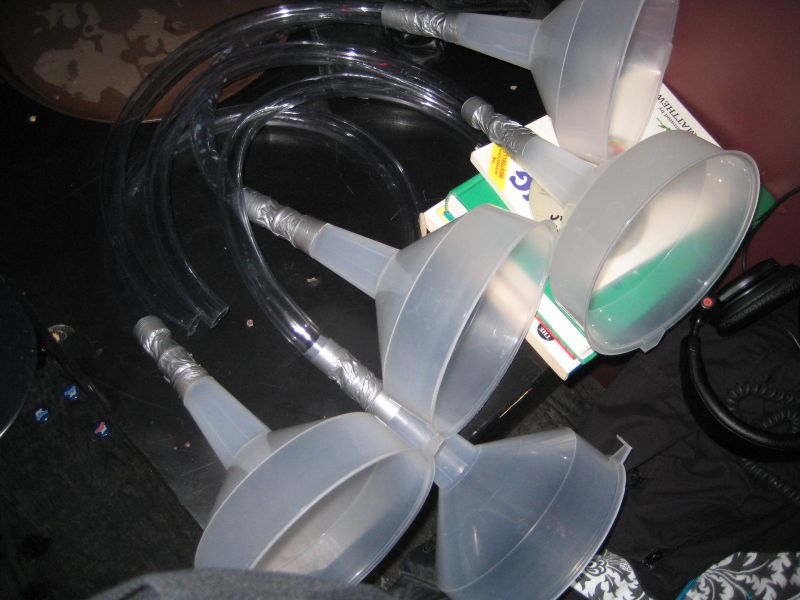The photograph features a close-up view of five beer funnels arranged side by side on a black table. Each funnel, fashioned from a clear plastic with a foggy appearance and a white brim, is connected to a highly transparent plastic tube using layers of silver duct tape. The scene is detailed with additional items scattered around the table, including a pair of headphones, some hardcover books in white and green, and a black tube with a spongy round piece attached. The setting also includes a background with a brown floor, a red cloth at one end, and a light and dark brown floral cloth nearby, adding depth and context to the arrangement of the beer funnels.